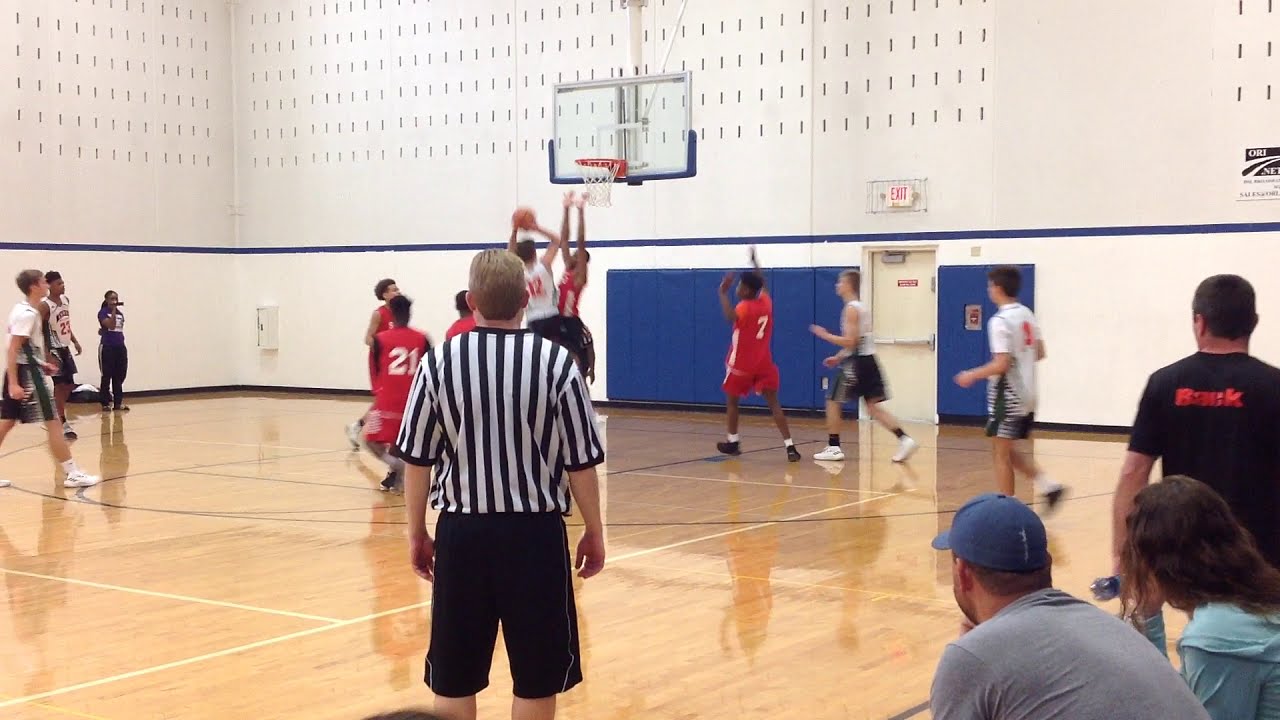The image captures an intense indoor basketball game on a shiny, light brown wooden court with clearly defined white and black lines. In the center forefront, a white referee with short, light brown hair, clad in a black and white vertically striped shirt and long black shorts, stands with his hands near his hips, his back turned towards the camera as he faces the players. Two high school-age teams are in action: one team in red jerseys and shorts, and the other in white jerseys with red numbers, blue accents, and navy blue shorts. Near the referee, a player wearing a red jersey with the number 21 appears ready to engage, while another player in a white jersey with the number 12 is visible to the right, and another in a red jersey with the number 7 stretches out their arm in a defensive move. In the background, a player in a white jersey is about to shoot the orange basketball, contending with an opposing player in red.

The game takes place in a gymnasium where the white walls are lined midway with blue mats for cushioning. An exit sign with a white frame and red lettering is visible behind a transparent basketball hoop, which features a prominent orange rim and a full net. There's an adjacent yellow door decorated with a red banner and white lettering. Spectators are gathered to the right side of the image; a man in a gray shirt and blue baseball cap leans forward attentively next to a woman with long brown hair wearing a light blue shirt. Standing beside them, a man in a black shirt with red lettering watches the game. The overall atmosphere is vibrant and engaging, reflecting the intensity and focus of both players and spectators alike.